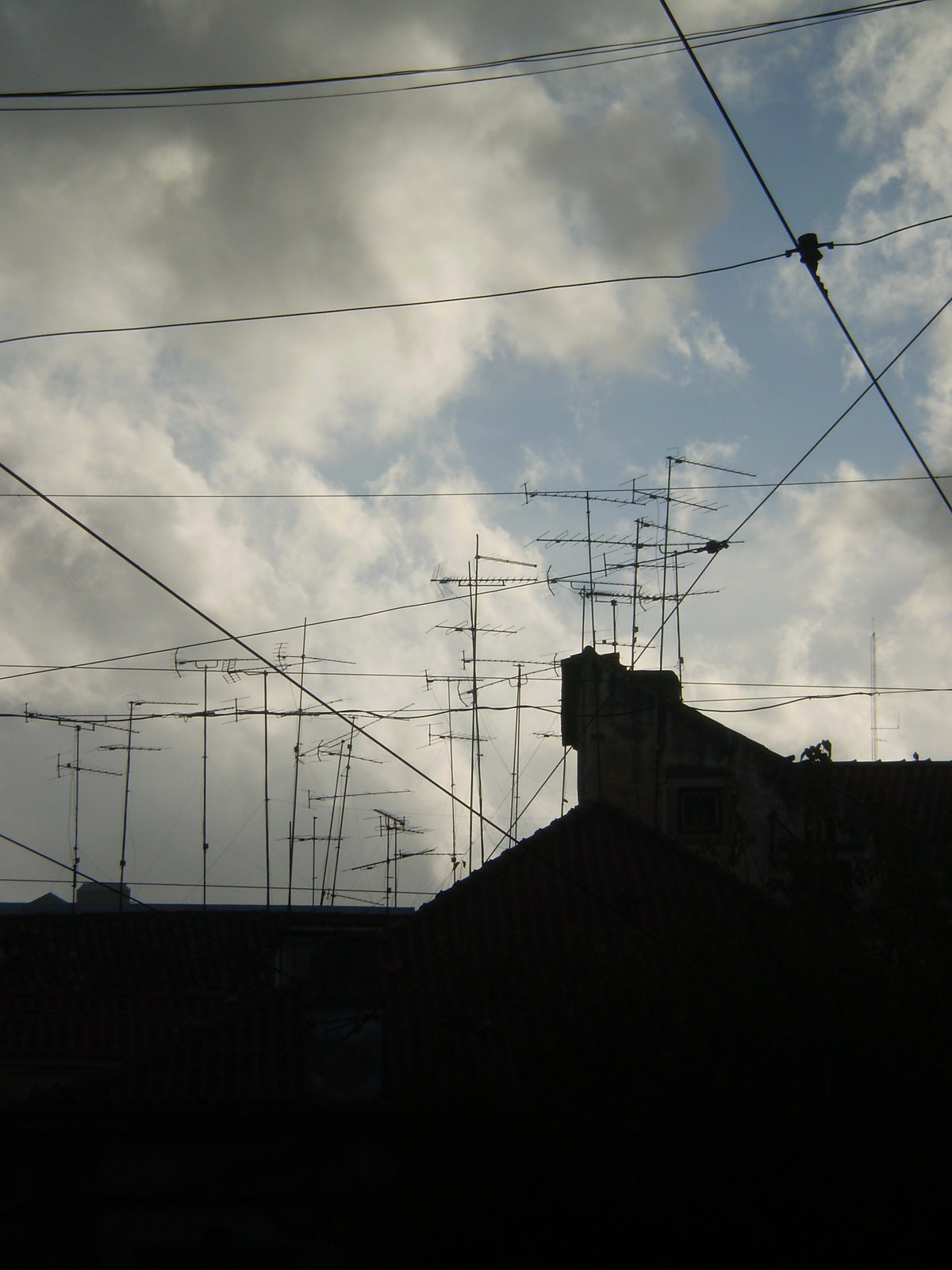The portrait-oriented color photograph encapsulates a striking scene at either dawn or dusk, where the interplay of light and shadow creates a dramatic atmosphere. The bottom third of the image is dominated by a complete black silhouette of several rooftops, suggesting a residential setting. Rising vertically just above this silhouette are various antennas used for TV reception, each differing in height and design; some feature thin single transmitters, while others have double protrusions with antennas extending horizontally to the left and right.

Interspersed among these antennas are a series of wires forming a somewhat haphazard lattice pattern, likely telephone lines, which crisscross across the sky and converge towards the rooftops. These wires, though not uniformly arranged, add an additional layer of complexity to the scene.

The backdrop of this silhouetted skyline is a mostly cloudy sky with a patchwork of gray and white wispy clouds. Notably, patches of blue sky are visible, particularly towards the upper right corner, providing a glimpse of clearer weather amidst the clouds. Some darker clouds, potentially rain-laden, are more prominent towards the top left, enhancing the image's moody yet captivating ambiance.